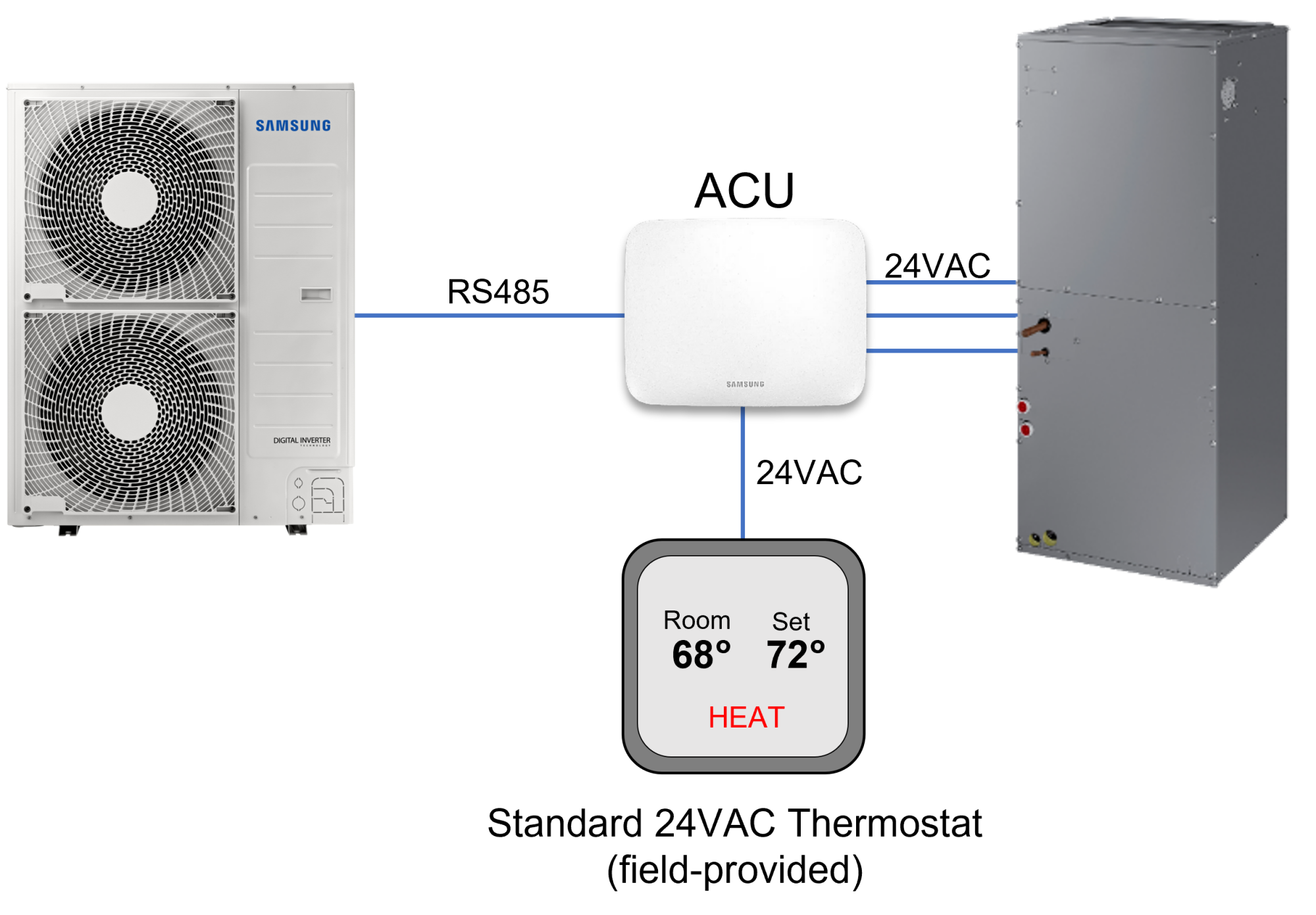This detailed infographic poster by Samsung showcases the functional components and connectivity of a 24 VAC thermostat, labeled as a standard field-provided unit. On the left side, two whirly fans are depicted, marked with the Samsung logo, and are connected by a blue line labeled RS 485 to a white control box in the center. This central box, labeled ACU (with portions of the letters SAM, SU, and G visible), is the primary control unit. From this ACU box, three white lines extend to the right, each labeled 24 VAC, connecting to a large industrial-looking metal cylinder structure. Additionally, a blue line descends from the ACU into a thermostat. The thermostat displays detailed settings: room temperature at 68 degrees, set temperature at 72 degrees, and 'heat' highlighted in bold red text. The thermostat area also features an annotation stating "standard 24 VAC thermostat (field provided)." The entire setup visually demonstrates the connectivity and operational procedure of the heating system, which is potentially a heat pump configuration.